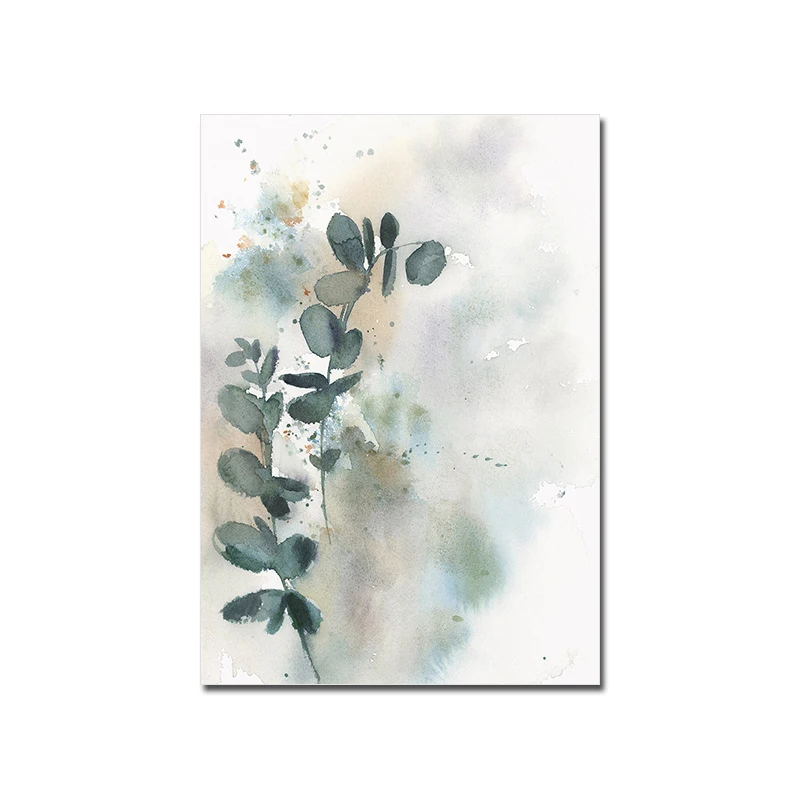The image is a watercolor painting on a white canvas, depicting simple, impressionistic eucalyptus leaves. The leaves, which are concentrated on two stems towards the left, showcase a gradient of greens from dark to light, and are detailed with subtle shading. The painting employs a bi-tone palette with greens, dark greens, lighter greens, and some accents of browns or orangey-browns. Additional specks of green, yellow, and hints of pink, blue, orange, tan, and purplish shades are dispersed throughout, adding depth and dimension, particularly smudged to the right side. The canvas is unframed and hangs on a wall, casting a shadow, giving the scene a refined yet simple appearance that could be mistaken for a photograph if not for its artistic perfection. The overall composition fades into the white canvas on the right, emphasizing the natural beauty of the eucalyptus leaves against a minimalist background.